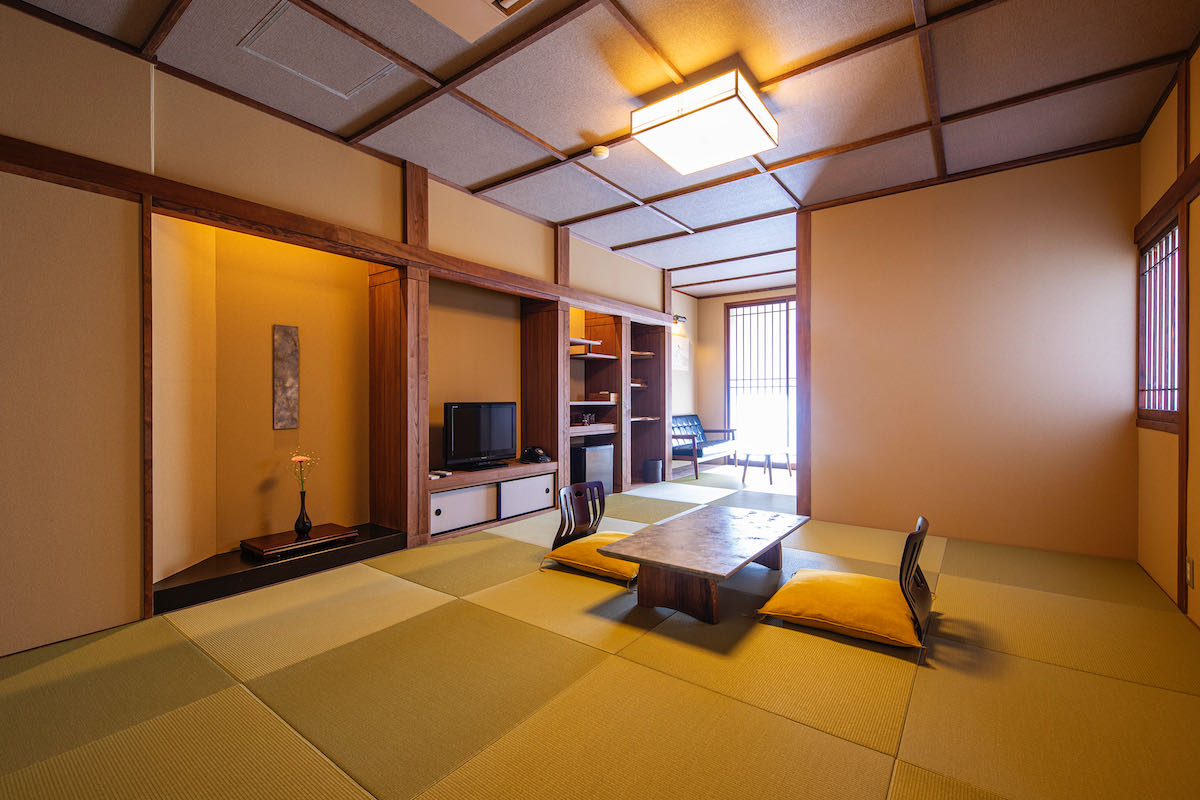The image depicts a cozy and oriental-styled living room with a significant focus on natural and earthy tones, creating a warm and inviting ambiance. At the center of the room, a low, brown wooden table with a gray and tan tabletop stands, designed for floor seating. Flanking the table are two legless chairs, each equipped with yellow pillows and brown wooden backs, characteristic of traditional Japanese dining. The floor features a mix of soft green, yellow, tan, and white square finishes that resemble tiles or carpet.

The room’s background includes several key furnishings: a black couch with brown legs, a black mini-fridge, and an array of shelves to the right of a black TV, which rests on white drawers within a brown cabinet. Additionally, a black vase with a white flower and a green stem is positioned in an indentation on the left wall, alongside some gray and tan artwork. The tan-painted walls are accented with dark brown wood trim, and a large window with shades allows rays of light to flood into the space, adding to the room's brightness and warmth.

The ceiling is white with brown wood accents and houses a yellow-lit fixture providing ambient lighting. Furthermore, a white device, likely for fire detection, is mounted on the ceiling, ensuring a blend of style and safety within the room. Overall, the room’s furniture and decor harmoniously blend traditional and modern elements, making it a functional yet aesthetically pleasing living space.